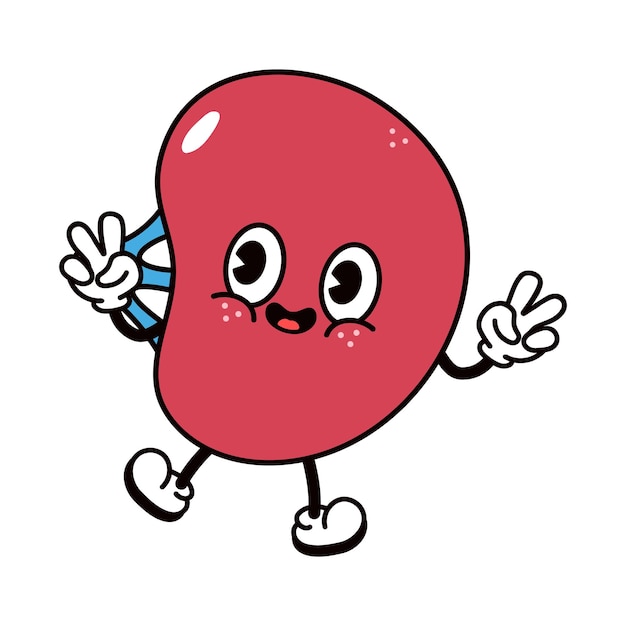The image is a color cartoon-style illustration featuring a jolly, bean-shaped character that might be a piece of bubble gum. The character is glossy and bright red, with large black eyes and prominent dimples that accentuate its cheerful expression. It has an open, smiling mouth, showcasing a red tongue. The character has two black arms ending in white-gloved hands, both of which are making the peace sign. It also has two black legs with white shoes. There are reflective spots and a white oval on its body, indicating a shiny surface. Behind the character’s right arm, there's a blue sticky substance resembling bubble gum, further hinting at its possible identity. The overall demeanor of the character is happy and lively, as if it’s in mid-motion, possibly laughing or talking.